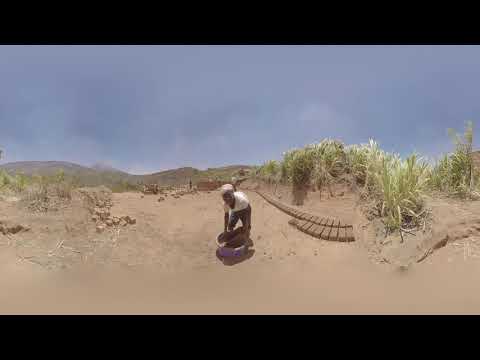The photograph, horizontally aligned and bordered with thick black bands at the top and bottom, depicts an arid, desert-like landscape reminiscent of Texas or Arizona. The sky above is mostly cloudy with bluish-gray and white hues blending together. In the distance, the outline of hilly terrain suggests vegetation-covered mountains or hills, anchoring the background. 

In the foreground, the sandy terrain varies from smooth at the bottom to disturbed, with visible footprints progressing towards the middle. Central to the image, an African-American man wearing a white short-sleeve shirt, shorts, and a hat, is slightly out of focus as he bends over, gripping a round object with a purple side. To his left, another person appears to be laying out rows of bricks, possibly letting them bake in the sun. Adding to the scene's texture, a wooden walkway extends into the distance behind the man, accompanied by tall grass emerging sporadically from the sand on the right side of the image. The overall setting is outdoors during the daytime, characterized by its dusty, sparsely vegetated environment. The colors prominent in the photograph are shades of brown, beige, white, black, green, and light blue.